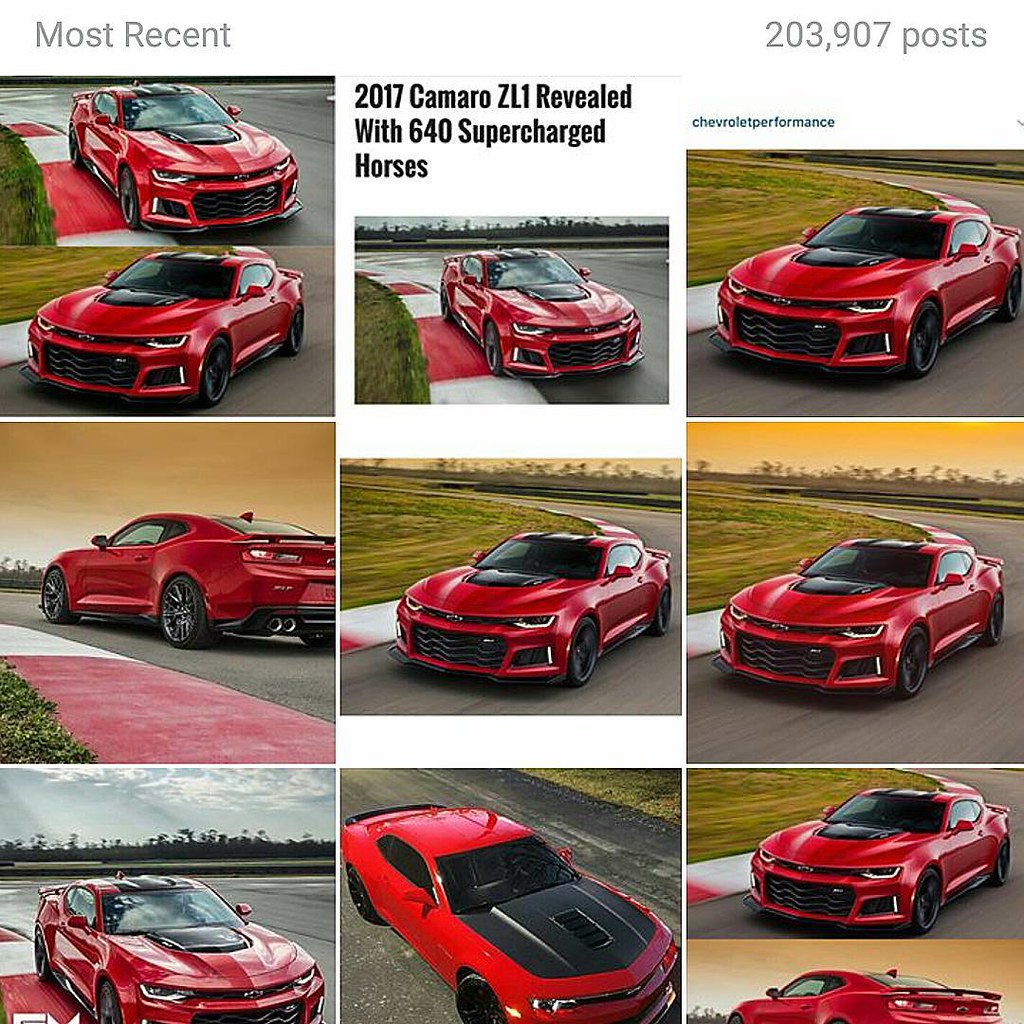This rectangular graphic features a collection of social media posts about the 2017 Camaro ZL1, organized in a window pane style format. At the top left, in gray text, it reads "most recent" and on the top right, it states "203,907 posts." The graphic is divided into three vertical columns.

In the left column, there are four pictures of a red Camaro taken from different angles. The center column starts with a header in black text on a white background that reads "2017 Camaro ZL1 revealed with 640 supercharged horses." Below this are three additional pictures of the red Camaro, with the bottom image featuring a unique detail: a completely black hood. The right column also displays four images of the same red Camaro, with the top right image captioned "Chevrolet Performance" in small print. Notably, the bottom image in this column is cut off at the wheels, appearing incomplete.

The Camaro is consistently depicted with a striking black racing stripe starting at the hood scoop, extending across the hood and roof. The images are well-spaced out, but none of the photos are particularly centered within the larger graphic. The various colors in the background and borders include red, black, white, gray, green, dark blue, yellow, and orange, contributing to the visual diversity of the composition.